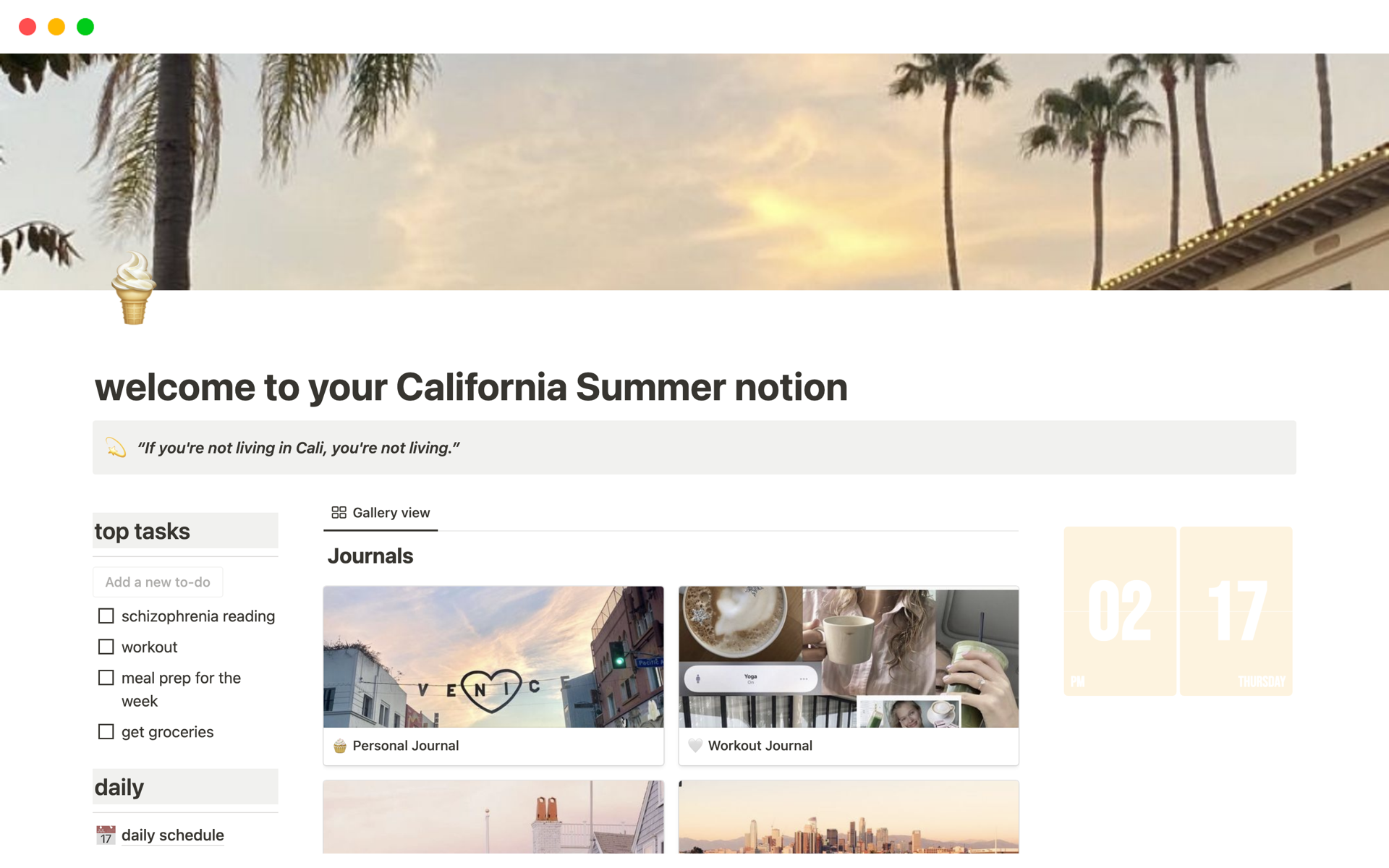The image showcases a Safari browser page with the header titled "Welcome to Your California Summer Notion." Dominating the top portion is a vibrant header image capturing an idyllic California scene featuring the sky, several palm trees, and the top corner of a building on the far right.

Beneath the header, prominent text declares, "If you're not living in Cali, you're not living." On the left side of the screen, there is a section for "Top Tasks" with four unchecked checkboxes labeled: "schizophrenia reading," "workout," "meal prep for the week," and "get groceries." Below this, there's an option to "add a new to-do" and a label for "Daily Schedule," accompanied by a calendar icon.

The primary section of the screen is labeled "Gallery View" under the heading "Journals." This section displays four images, although only the top two are fully visible. The first image, captioned "Personal Journal," is displayed under a banner with the word "Venice," likely referring to Venice, California. The second image, labeled "Workout Journal," seems to be a collage incorporating elements such as a coffee cup, a woman holding a coffee cup, and another woman holding a smoothie. The bottom two images are partially obscured by the edge of the screen, leaving their captions hidden.